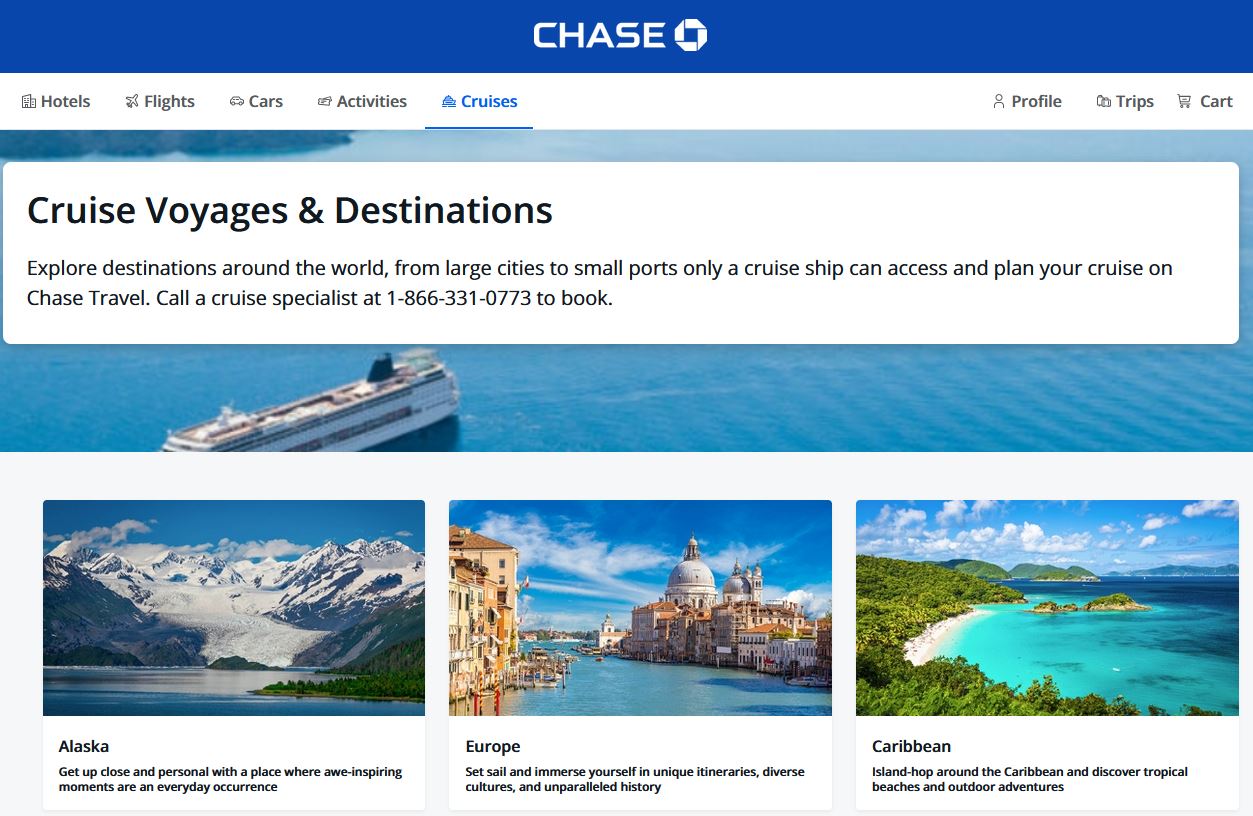This image taken from the Chase website features a prominent Chase emblem, characterized by a square logo with a white circle elegantly surrounding it. The upper section of the webpage is dominated by a royal blue rectangle that houses the "Chase" name. Below this is a white navigation bar listing various travel options: "Hotels" on the left, followed by "Flights," "Cars," "Activities," and "Cruises," with "Cruises" being underlined, indicating it is the selected option. 

To the right of this bar, the white space continues with links labeled "Profile," "Trips," and "Cart." Below the navigation bar, the central area of the page displays a scenic image of a waterway featuring a cruise ship along with the text "Cruise Voyages and Destinations." This section invites users to "Explore destinations around the world from large cities to small ports only a cruise ship can access," encouraging them to plan their cruise through Chase Travel. It also provides a phone number to contact a cruise specialist for bookings.

At the bottom of the screen are three picturesque images showcasing potential cruise destinations. The first image on the left depicts the breathtaking landscapes of Alaska, featuring massive snowy mountains. The middle image illustrates Europe, presenting an iconic waterway bordered by historic buildings. The third image on the right highlights the Caribbean, displaying crystal-clear teal waters and lush greenery. Each image entices viewers with the distinct allure of these renowned travel destinations.